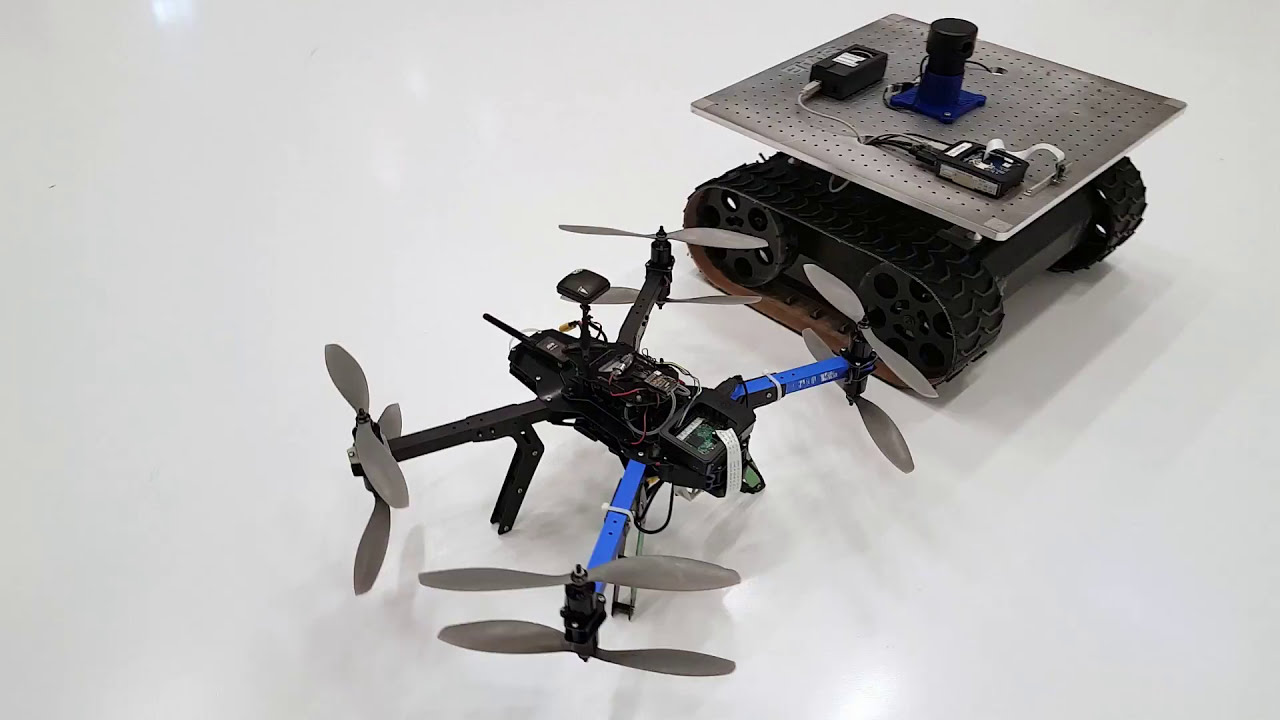This image showcases a modified, do-it-yourself black and blue drone and a rover-like remote-controlled tank situated on a shiny white table. The drone features four arms, the rear ones in blue and the front in black, each equipped with a set of four gray propellers. It rests on four stands for stable grounding when not flying, and various wires and components are visible on its body, including a possible antenna. To the upper right of the drone, the tank-like rover has black rubber treads wrapping around wheels with distinctive circular holes. The rover's silver metal plate, perforated with numerous holes, supports an array of bolted-on electronics, including a motor, battery pack, and something resembling a computer, along with possible controllers or a joystick, hinting at its adaptable functionality.